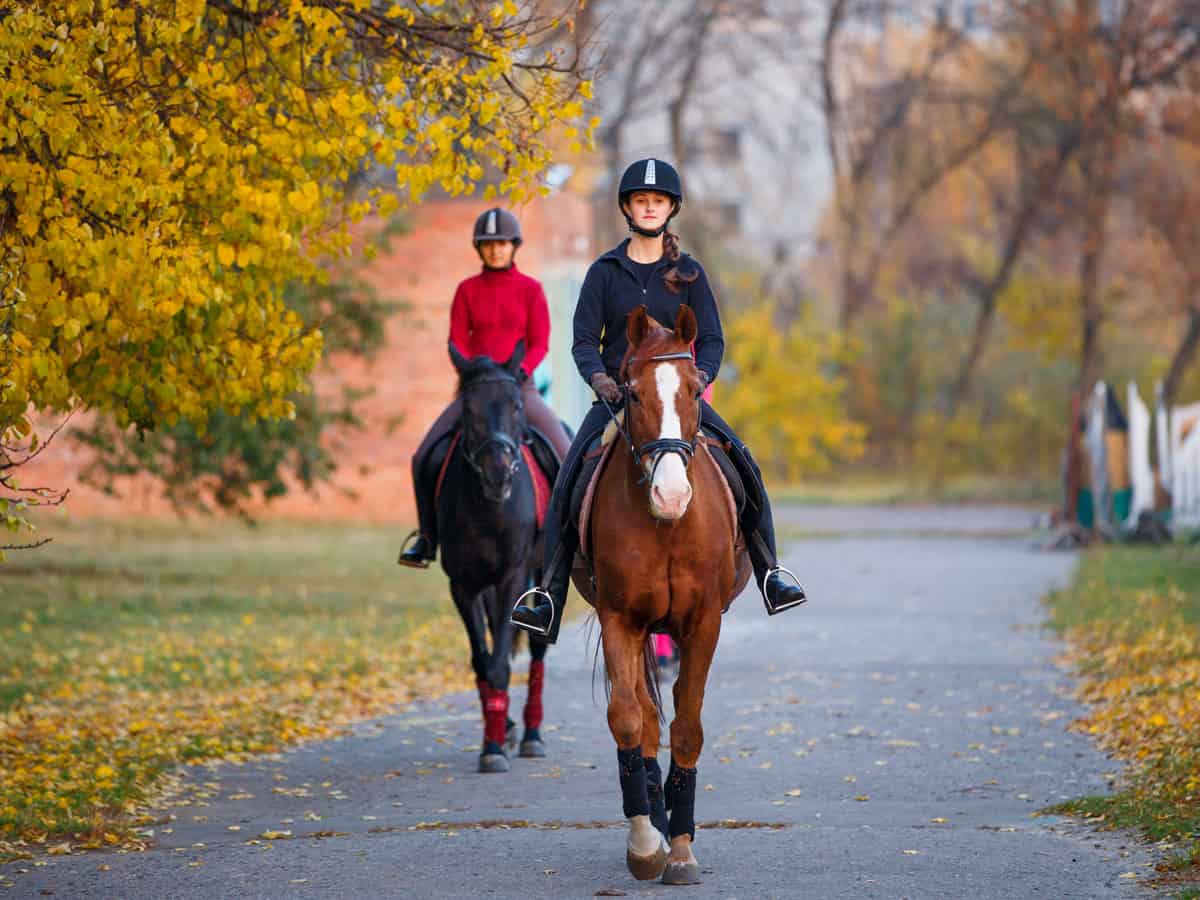Here is a detailed consolidated caption based on the voice captions provided:

In this outdoor daytime photograph, we see two individuals riding horses along a wide paved pathway in a park during the fall season. The pathway, surrounded by grass and trees with yellow leaves, some of which have fallen to the ground, suggests a serene autumn setting. 

To the right, in the forefront, is a reddish-brown horse with a distinctive white muzzle and stripe down its face. The horse has perked ears and black markings, or socks, on its legs between the knees and hooves. The rider, who appears to be a teenage girl, is dressed in a blue helmet, a matching blue zip-up hoodie, and blue pants.

To the left and slightly further back is a dark-colored, black horse with its ears pulled back and wearing red protective leg gear. The rider is clad in a brown helmet, a red long-sleeved jacket, and brown pants. The scene captures the tranquil yet lively essence of horseback riding in a picturesque park during autumn.